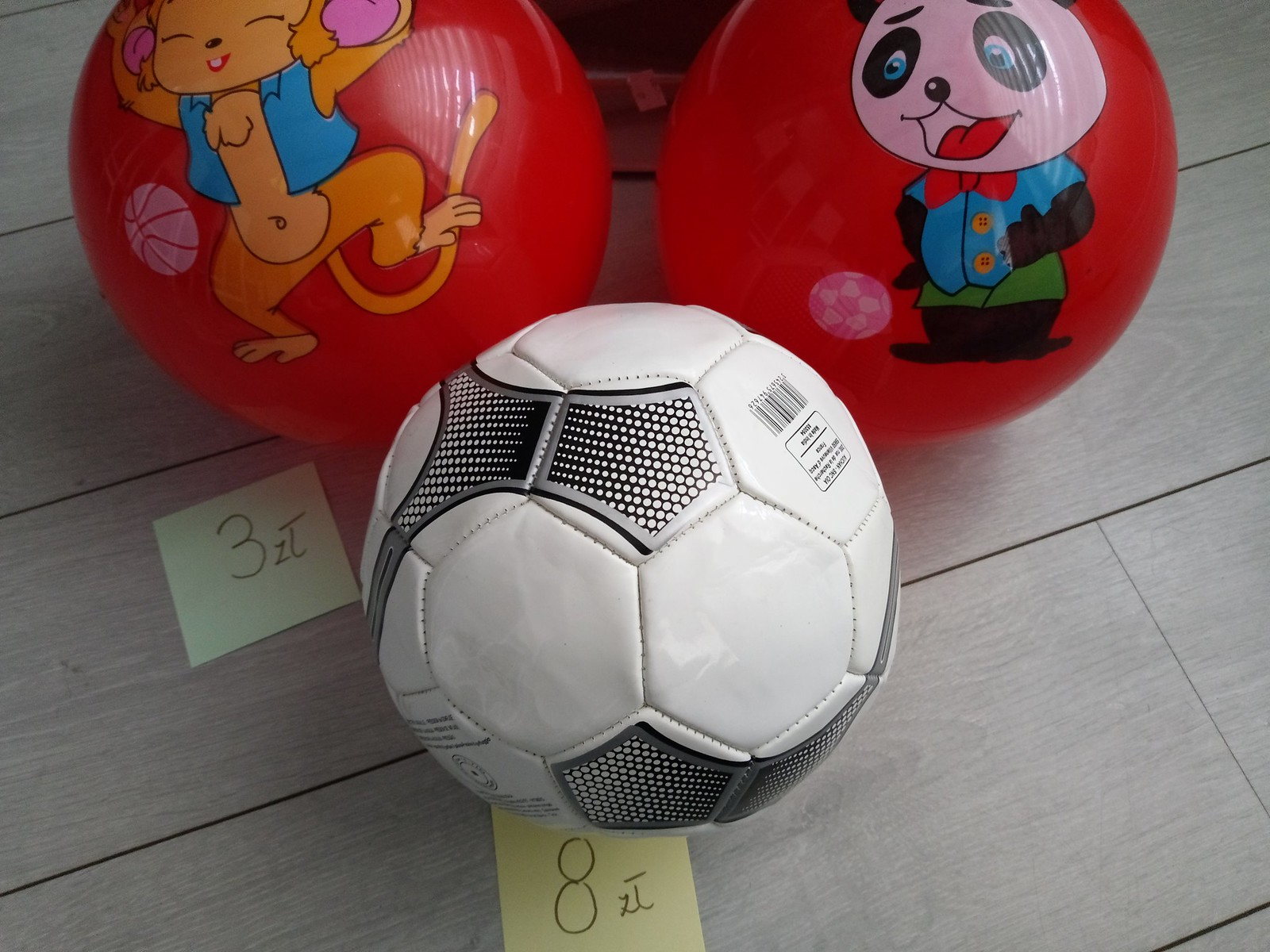This color photograph features three children's balls arranged in an upside-down triangle formation on an ashen, wood grain print, synthetic wood floor. The prominent black and white soccer ball, resting at the bottom in the foreground, is adorned with hexagonal panels and black and silver trim. One side of the soccer ball shows a barely readable label and a barcode. Above the soccer ball are two bright red play balls, each featuring playful cartoon characters. The ball on the upper left displays a light brown mouse with closed eyes, dressed in a blue sleeveless vest and dancing joyfully. On the upper right, the red ball depicts a panda bear with a big round face, blue eyes, a red bow tie, a blue shirt, and green shorts, appearing animated and cheerful. Both red balls also feature a small printed soccer ball within their designs, enhancing the playful soccer theme of the photograph. Additionally, stickers labeled with the numbers "3" and "8" can be seen on two of the balls.